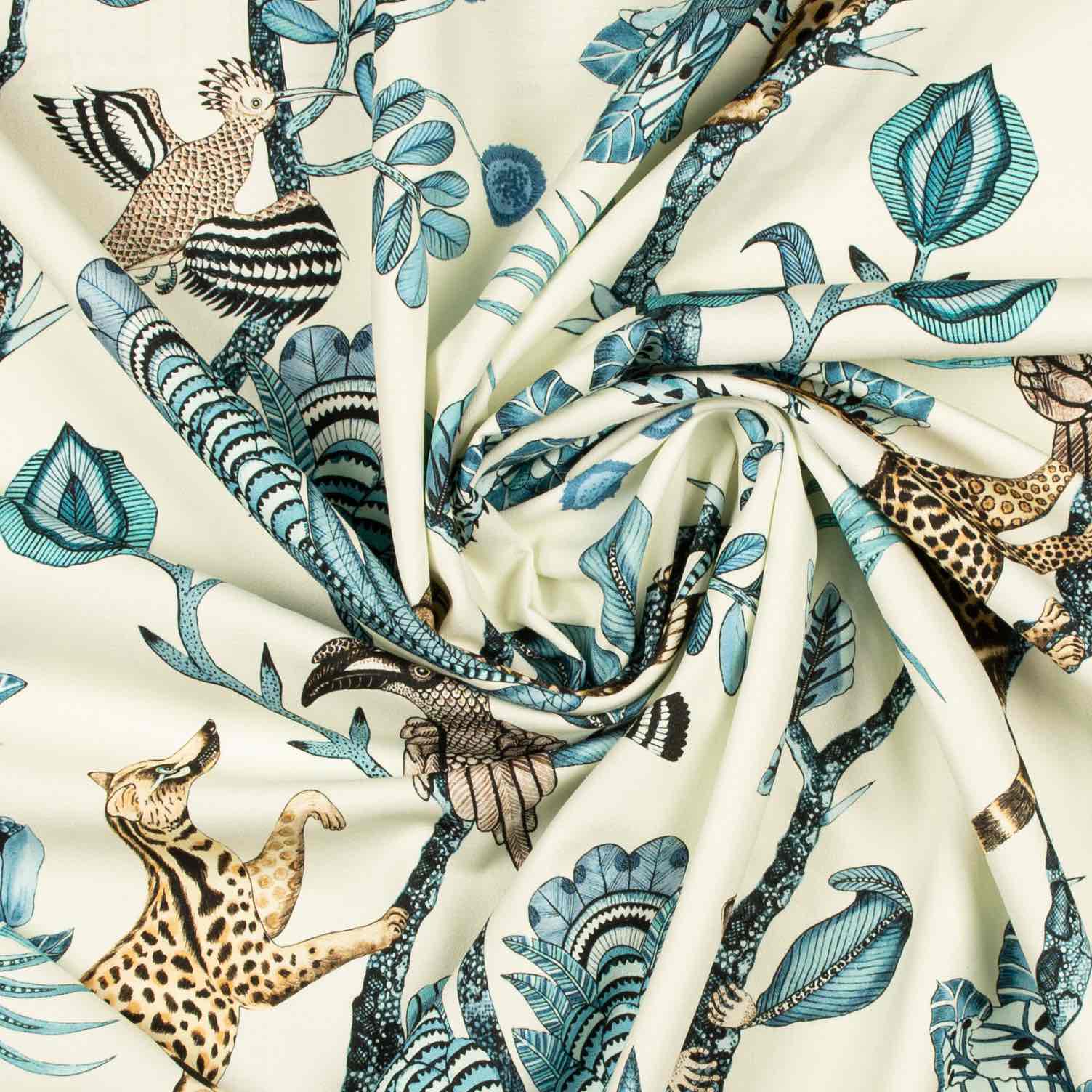This detailed, close-up color photograph captures a piece of fabric that fills the entire square frame. The fabric appears to be thin, possibly a blanket or tablecloth, and is gathered and twisted at the center, creating folds. The background of the cloth is white, adorned with a vibrant pattern of animals and botanical elements in shades of blue, brown, and black. Notably, the fabric features a variety of animals, such as a spotted cat resembling a cheetah or ocelot, a pheasant-like bird in flight, a distinctive toucan near the center, and possibly even a giraffe-like figure. Interspersed among these creatures are blue leaves, flowers, and tree limbs with tribal designs, enhancing the jungle or nature-themed aesthetic. The pattern appears to repeat consistently across the fabric, giving it a rich and complex visual texture.